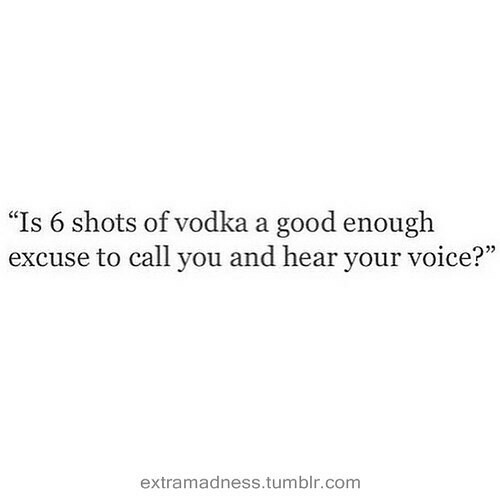The image features a minimalist design with black text on a white background, utilizing a serif font likely to be Times New Roman. In the center of the image, positioned in two distinct lines and enclosed in quotation marks, is the quote: "Is six shots of vodka a good enough excuse to call you and hear your voice?" The text is formatted with the number "6" instead of the word, and the first letter "I" is capitalized. At the very bottom of the image, written in a lighter gray sans serif font, is the source link "extramadness.tumblr.com," serving as a faint watermark. The image is stark and uncluttered, emphasizing the quote and its origin without any additional elements.